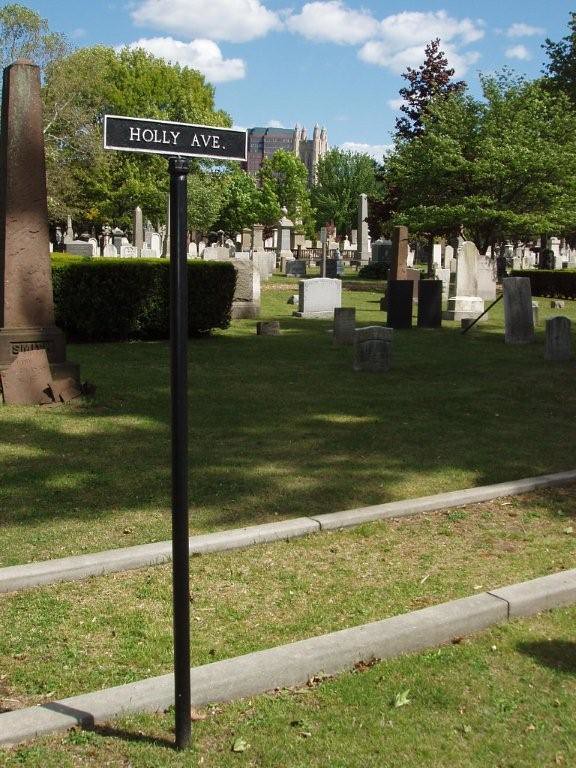The image captures a serene cemetery scene under a blue, partly cloudy sky. In the foreground stands a black post with a rectangular, black sign outlined in white, reading "Holly Avenue" in white lettering. The cemetery is vast, with well-maintained grassy ground covered with scattered leaves. White, black, gray, and even some brown gravestones and headstones of various shapes and sizes, including ornate and tall obelisks, are prominently visible. To the left, there is an additional brown structure or design adding to the scene's complexity. The background features lush green trees, and beyond them, the top of a very tall building can be seen, further highlighting the serene yet urban setting of the photograph.